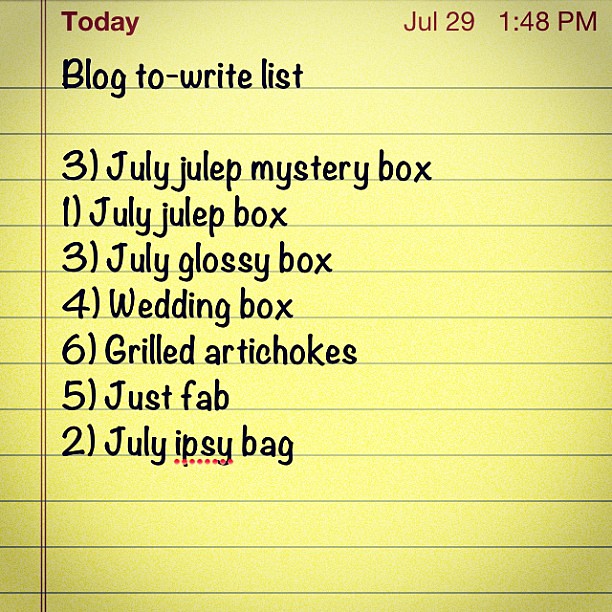The image depicts a digitally synthesized yellow notepad, resembling the old iPhone Notes application. Blue horizontal lines evenly spaced from right to left structure the background, while a double vertical red line on the left forms a slim column. At the top left, "Today" is written in dark red text, followed by the date "July 29" and the time "1:48 p.m." in the same red color at the top right. Below "Today," a to-do list is written in black text on individual blue lines. The list reads:
1. "Blog to write list"
2. "3.00 July Julep Mystery Box"
3. "1.00 July Julep Box"
4. "3.00 July Glossy Box"
5. "4.00 Wedding Box"
6. "6.00 Grilled Artichokes"
7. "5.00 Just Fab"
8. "2.00 July Ipsy Bag"

Each item is aligned to the right of the numbers, with capitalized first letters and no periods.